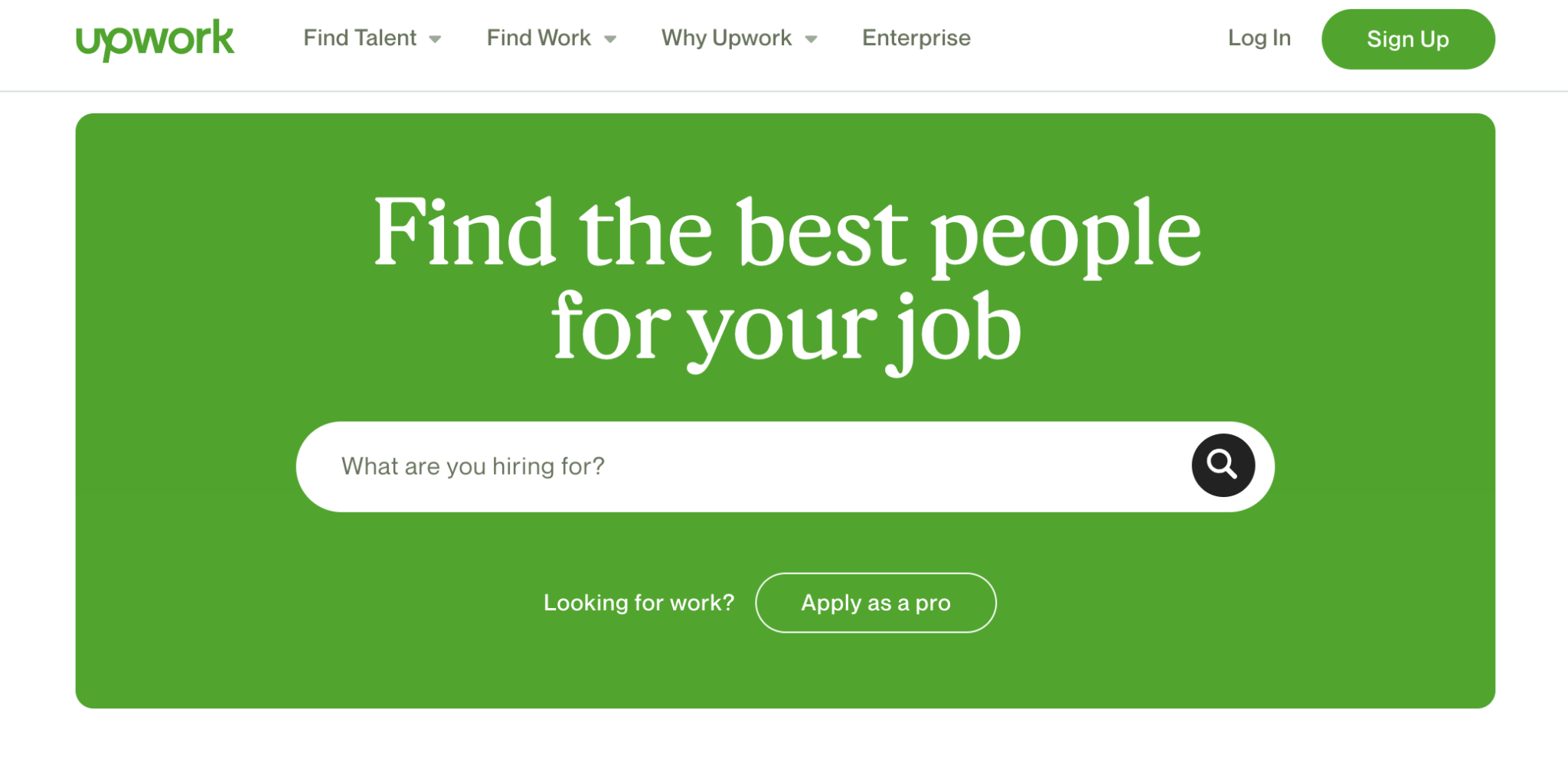The homepage of the Upwork website is well-structured and visually appealing, showcasing a green-themed color palette consistent with its logo. Across the top navigation bar are several menu options, including "Find Talent," "Find Work," "Why Upwork," and "Enterprise." In the upper right corner, users can find "Login" and "Sign Up" options, with the "Sign Up" button highlighted by a green background.

Dominating the central portion of the page is a large green section with prominent white text that reads, "Find the Best People for Your Job." Below this header, there is a search bar accompanied by the prompt "What are you hiring for?" in black or gray text, alongside a black magnifying glass icon on the right. Beneath the search section, there's a call-to-action element for job seekers that says "Looking for Work?" followed by an oval-shaped button labeled "Apply as a Pro." This section indicates that professionals can apply to offer their services on the platform, while clients can search for specific talents, such as photographers, to meet their needs. Overall, the page efficiently guides both freelancers and clients to the resources they require. Transcribed by https://otter.ai